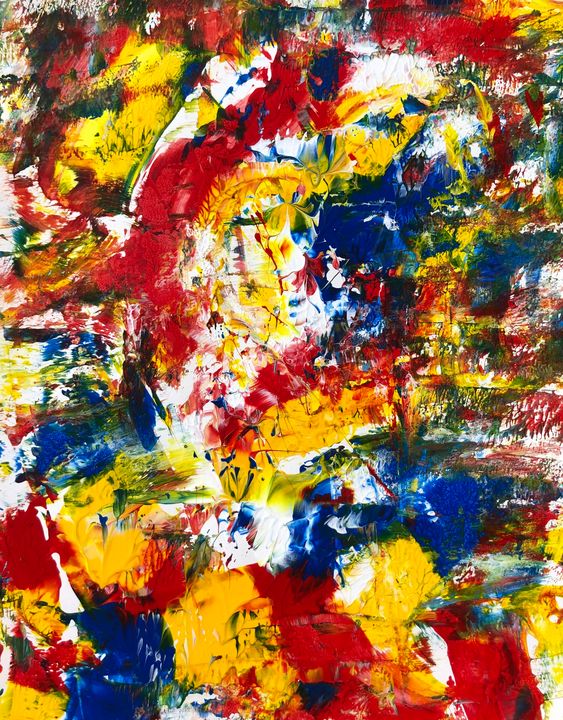This image captures a rectangular artistic painting that features vibrant, abstract strokes of red, yellow, blue, and green paint. The composition is spontaneous and freeform, lacking a discernible pattern or subject, which gives it a tie-dye-like appearance. Various brush strokes and swabs of paint overlap and blend, creating a dynamic interplay of colors. The green hues appear to result from the natural mixing of the primary colors. The overall effect is a lively and colorful mosaic, evoking a sense of playful creativity.